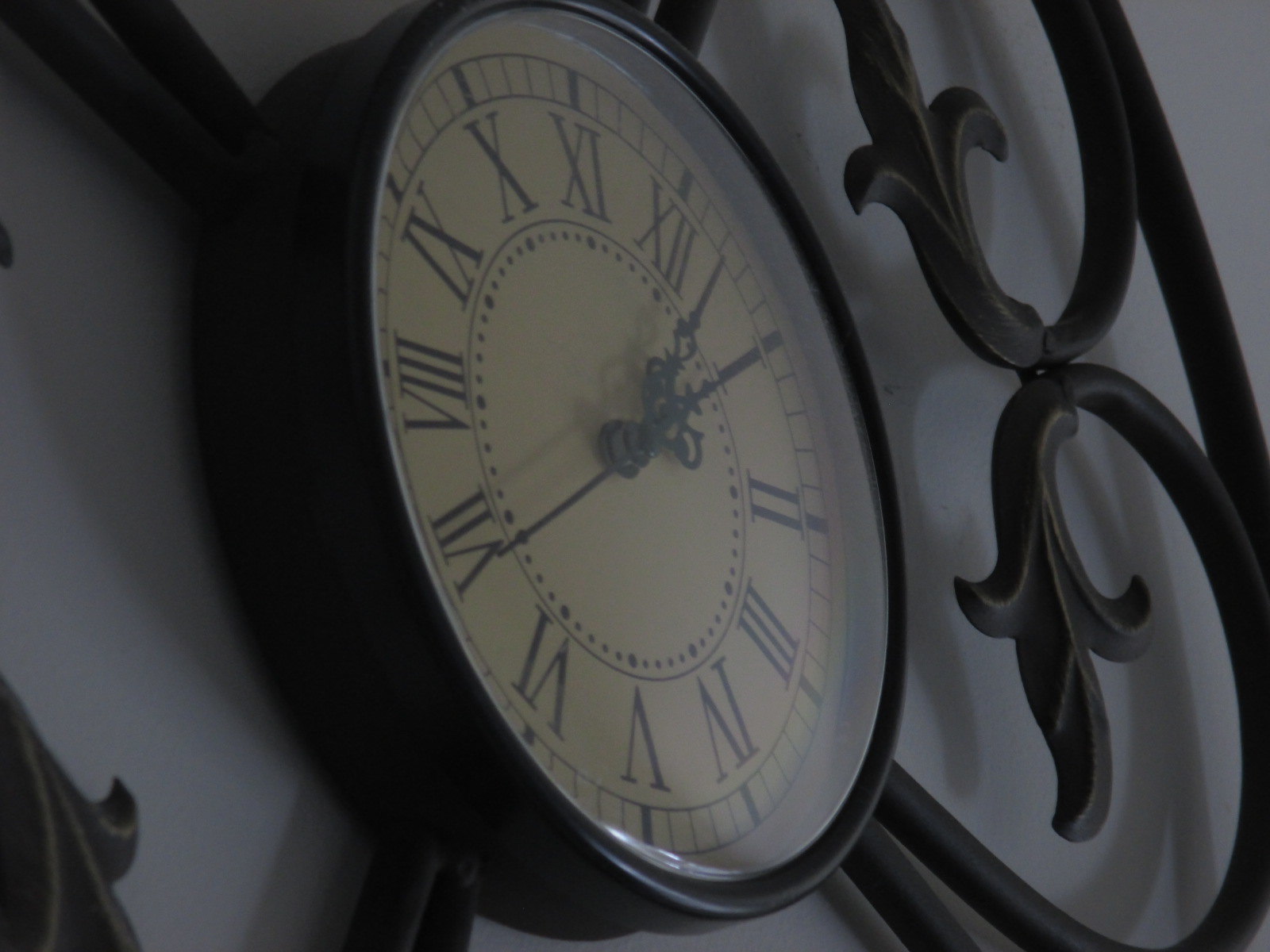The image features an elegant, analog clock with a sophisticated design. The clock's central face has a warm yellow-beige background set within a sleek black frame. Black Roman numerals elegantly mark the hours, and the ornate black hour and minute hands resemble spears with intricate tips. The clock is bordered by a decorative metal framework, fashioned into artistic branches ending in trident-like leaves, all in a matching black color. This artistic metalwork casts subtle shadows on the plain white wall behind it, adding depth to the composition. A clear glass or plastic pane covers the clock face, contributing to its refined appearance. The clock and its decorative frame are partially visible from a left-sided angle, enhancing the image's three-dimensional effect.